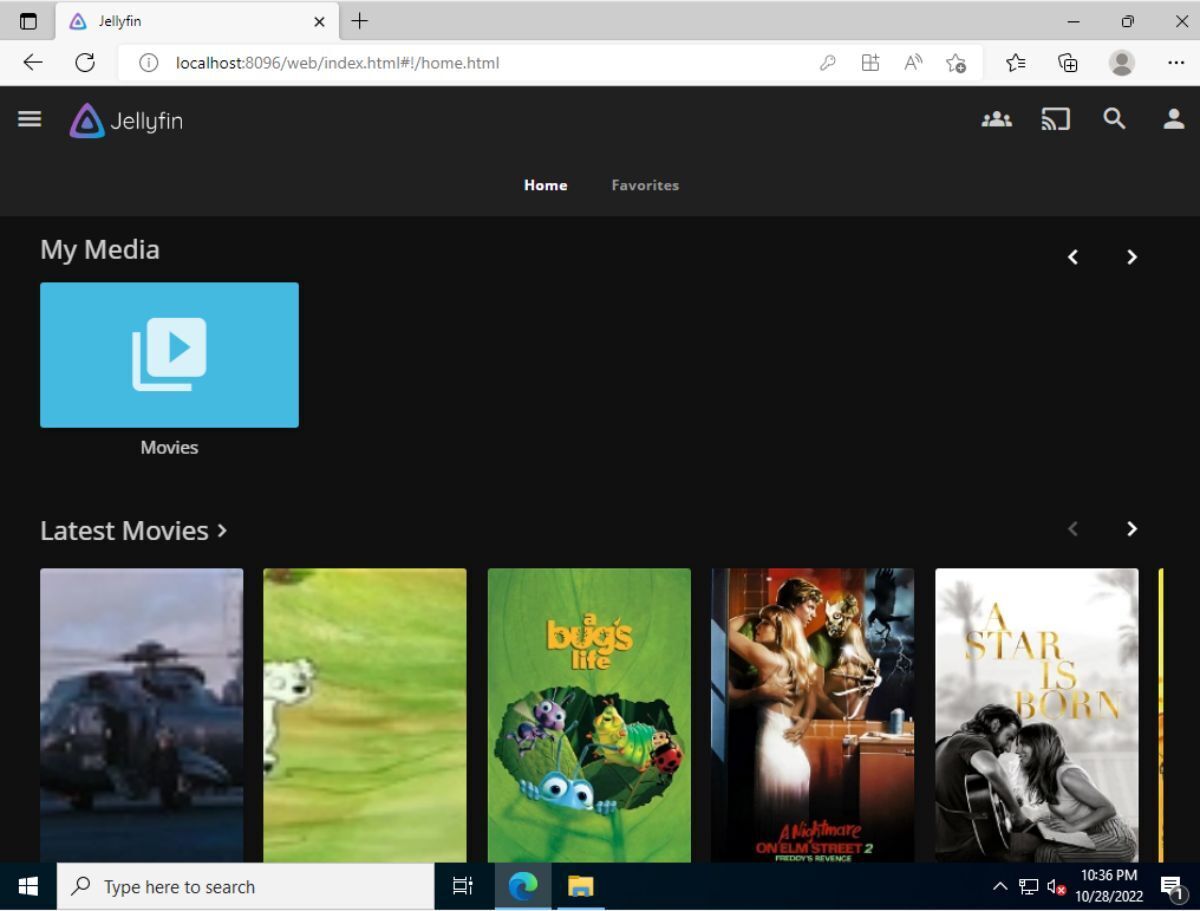This is a detailed screenshot from the Jellyfin website, showcasing a user's movie library. The main section of the page features a sleek black background displaying the covers of five selected movies from the user's collection. 

**Top Navigation Bars:**
1. **First Bar:**
   - **Gray Search Bar:**
     - Search query "Jellyfin" entered.
     - An 'X' icon to clear the search.
     - Interface control icons including minimize (-), maximize (□), and close (X) on the right.
2. **Second Bar:**
   - **Navigation Controls:**
     - Left arrow for back navigation.
     - Refresh arrow.
   - **Address Bar:** 
     - Displays "localhost:8096/web/index.html-home.html."
   - **Icons:**
     - A series of eight icons on the right, including tools, fonts, and profile settings.

**Website Header:**
- **Top Left:** 
  - Jellyfin logo, featuring a gradient triangle with a teardrop shape in purple and blue.
  - "Jellyfin" written in white font.
- **Top Right Icons:**
  - People icons, Movies, a Search icon, and Profile icon.

**Main Content:**
- **Tabs:** 
  - "Home" is selected, with another tab for "Favorites."
- **Section Title:** 
  - "My Media" with a blue box containing a white arrow pointing right.
  - Underneath, the section titled "Movies."
- **Displayed Movies:**
  1. A movie cover showing a military helicopter grounded with its blades rotating.
  2. A field scene featuring a Dalmatian, resembling the cover of "101 Dalmatians."
  3. The cover of "A Bug's Life," depicting leaves and five cartoon bugs.
  4. A romantic scene with a man and woman embracing.
  5. A man playing a guitar with a woman leaning towards him, representing "A Star is Born."

**Footer:**
- **Additional Search Bar:**
  - Positioned at the bottom.
- **Right Side:** 
  - Time displayed as 10:36 PM.
  - Date shown as 10/28/2022.
  - Various standard icons typical in a Windows navigation bar.

This detailed screenshot encapsulates the Jellyfin interface, providing a comprehensive view of the user's movie viewing options and various navigation elements of the website.